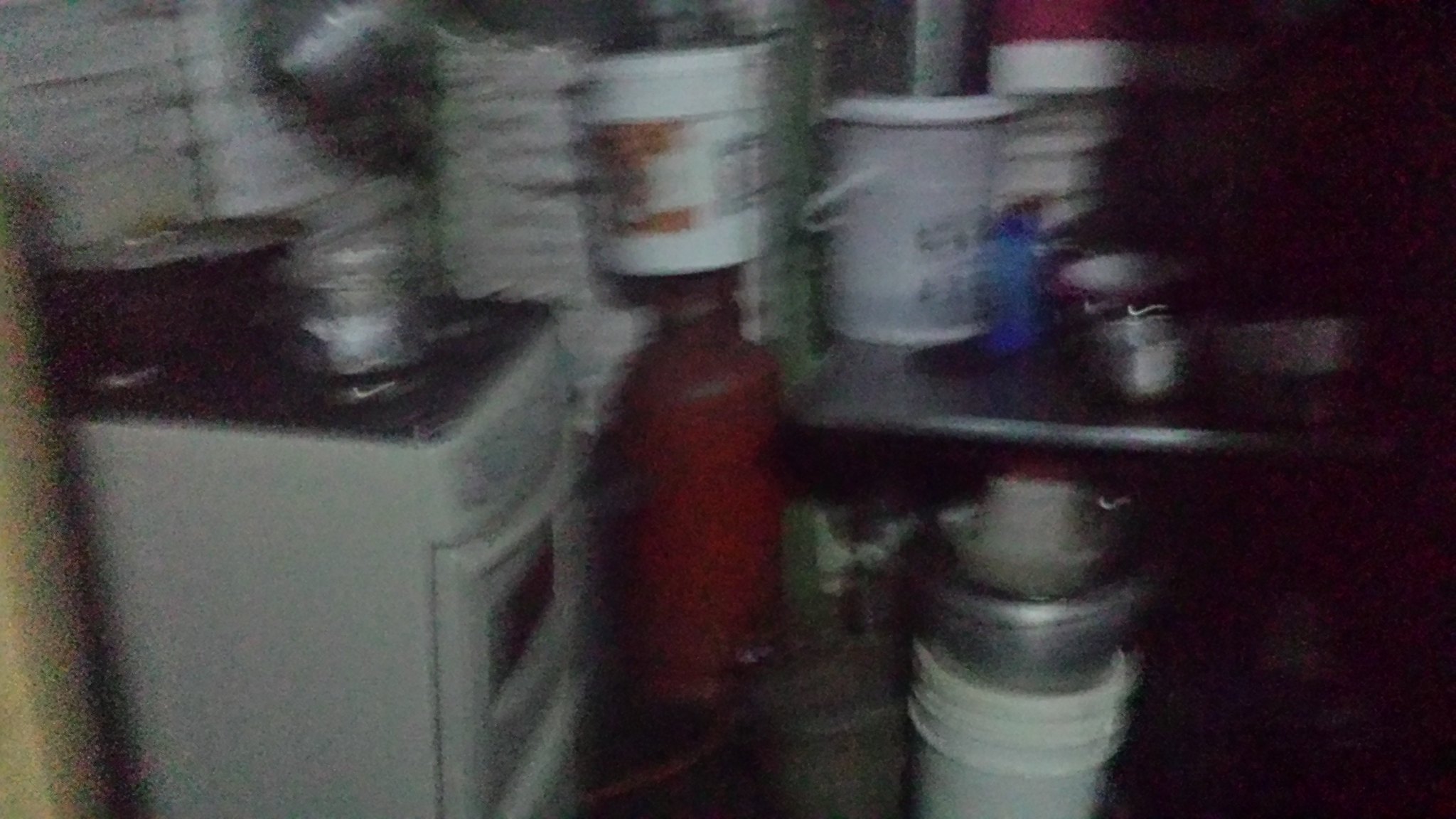The image is a very blurry, low-quality photograph of what appears to be a cluttered basement or kitchen space, shrouded in darkness and lacking sufficient lighting. On the left side, there is an old white stove with a black top, barely discernible dials, and an oven door handle. Atop the stove, there are several items, including paint-like cans. Adjacent to the stove on the right is a solid red cylinder, possibly a propane tank, topped with a white bucket. Extending to the right of the frame is a metal table cluttered with more white barrels, pots, and pans. Underneath this table, additional pots, buckets, and a bowl are precariously stacked. The overall scene suggests a storage or possibly a commercial kitchen area, characterized by its disarray and the various cooking and storage items scattered throughout.